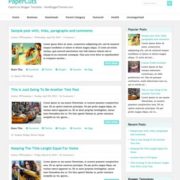This image displays a small, zoomed-out screen featuring a layout typical of a web page. At the top, there is a title highlighted in blue, followed by seven distinct categories arranged directly underneath. Below these categories, the main content area presents three article titles, each accompanied by a brief summary that remains too small or blurred to read clearly. These articles are arranged in a vertical sequence with a top, middle, and bottom position. On the right-hand side of the screen, there is a "Popular" section showcasing three additional articles in a more compact format. Beneath this section, there are three to four website links, displayed in a light blue color. The background of the majority of the image, approximately 80%, is light gray, while the top portion consists of a white background.